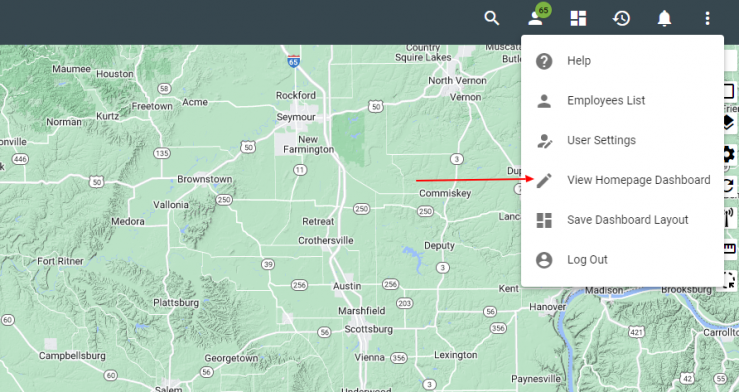A detailed map of an area in the United States is displayed on a screen, featuring Austin and Rockford prominently. The map shows highway I-65, part of the Eisenhower Interstate Highway System, running through the area. The central terrain appears mostly flat, while the regions to the left and right reveal slight elevations, giving a more mountainous appearance. 

At the top of the map, a dark background bar is visible, containing various interface icons, including a magnifying glass for search functionality and a profile picture icon marked with a badge displaying '65', possibly indicating unread messages or notifications. Additional icons present include one resembling an alarm, likely for notifications.

Moreover, a drop-down menu is open, highlighting several options such as 'Help', 'Employees List', 'User Settings', 'View Homepage Dashboard', 'Save Dashboard Layout', and 'Logout'. An arrow points specifically to the 'View Homepage Dashboard' option. On the map, a river can be seen on the right side, with the city of Lexington mentioned nearby.